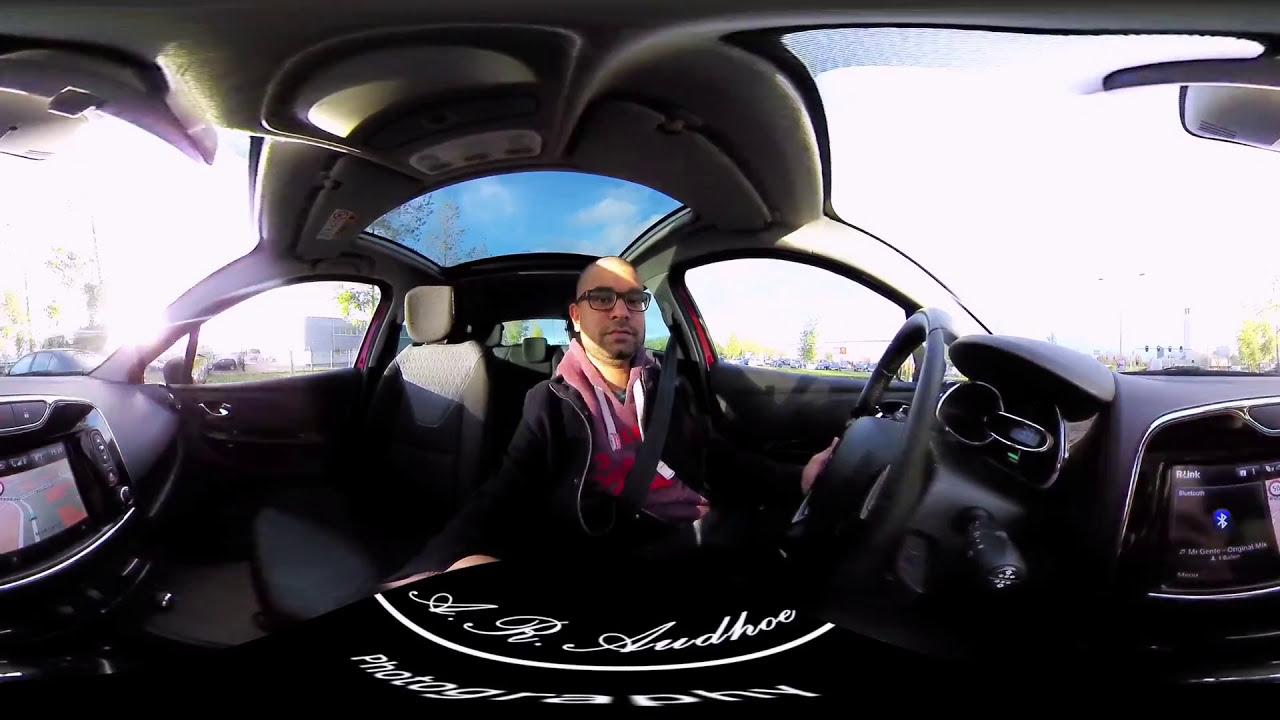The image depicts a man with extremely short hair, almost bald, and a slight beard or goatee, sitting in the driver's seat of a car. He is wearing glasses with black frames and a burgundy hoodie with some unreadable writing on it, layered underneath a black unzipped jacket. His left hand is resting on the black steering wheel and his right hand appears to be holding the camera, suggesting he is taking a 180-degree panoramic photo from inside the vehicle. The car's roof is gray and features a large sunroof through which a clear blue sky with a few small white clouds is visible. The dashboard is visible, showcasing a small GPS screen displaying a road map and other information like Bluetooth connectivity. It is a bright and sunny day outside, as indicated by the vivid light coming through the windows, revealing several trees, traffic lights, and a house with a parked car in the distance. The bottom of the image is labeled with "A-R-A-U-D-H-O-E photography".